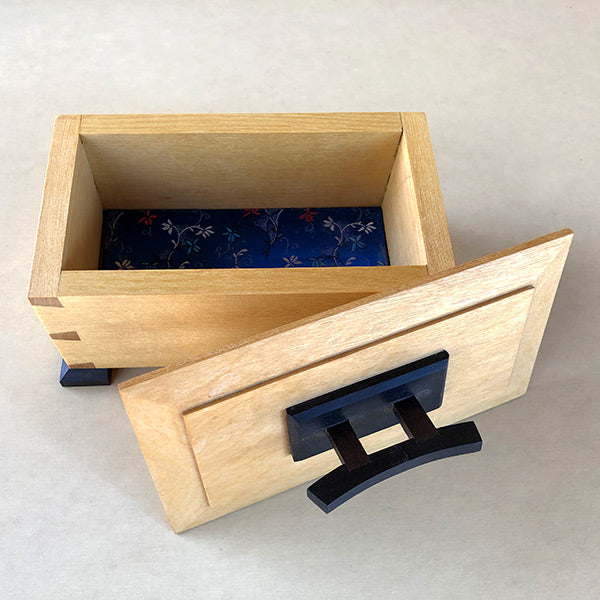This is an overhead photograph of a small, rectangular wooden box with thick sides, positioned on a textured white countertop. The box features short, black, angled feet that appear to be made of metal. Inside the box, at the bottom, there is a piece of shiny dark blue fabric adorned with white and red flowers and green stems. In the bottom left corner of the box, three lines indicate where different pieces of wood join together. Leaning against the bottom right corner of the box is its lid, which matches the box's light tan wood. The lid has a curved black metal handle fixed to its center. The scene is set in a way that showcases the box, highlighting its interior and detailed craftsmanship.